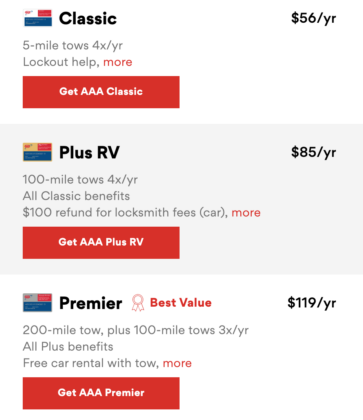The image displays three subscription options for Triple A, organized in a vertical stack.

**Option 1:**
- **Title:** Classic (Located at the top left corner)
- **Price:** $56 a year (Located at the top right corner)
- **Benefits (in light gray font):**
  - 5-mile tows, four times a year
  - Lockout help
  - More (in red font, likely a clickable link for further details)
- **Button:**
  - A red rectangular button that says "Get Triple A Classic" in white font

**Option 2:**
- **Title:** Plus RV (Bold black font, located on the left side)
- **Price:** $85 a year (Located on the right side)
- **Benefits (in light gray font):**
  - 100-mile tows, four times a year
  - All Classic benefits
  - $100 refund for locksmith fees
  - Car rental benefits
  - More (in red font, likely a clickable link for further details)
- **Button:**
  - A red rectangular button that says "Get Triple A Plus RV" in white font

**Option 3:**
- **Title:** Premier (Bold black font, located on the left side)
- **Label:** A small red ribbon next to the title that says "Best Value" in red font
- **Price:** $119 a year (Located on the right side)
- **Benefits (in light gray font):**
  - 200-mile tow, plus 100-mile tows, three times per year
  - All Plus benefits
  - Free car rental with tow
  - More (in red font, likely a clickable link for further details)
- **Button:**
  - A red rectangular button that says "Get Triple A Premier" in white font